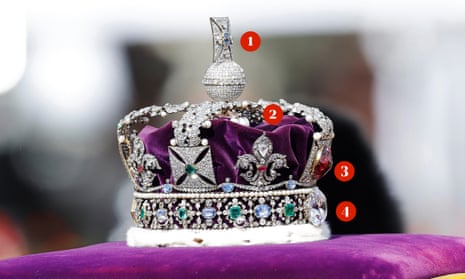This image portrays a majestic royal crown, reminiscent of those worn by the kings and queens of England. The crown, decorated with an array of splendid jewels, including diamonds and richly colored deep turquoise stones, is perched regally on a plush purple velvet pillow. The crown itself is crafted from silver and features an intricate combination of decorative elements such as a German cross composed of four triangles forming a square, several fleur-de-lis shapes, and a large brilliant diamond positioned just above the base.

The interior of the crown is lined with luxurious purple velvet that matches the pillow beneath it. The base is trimmed with white fur, adding to its opulent appearance. At the top of the crown sits a mirrored sphere adorned with additional jewels, enhancing its grandeur. Surrounding the crown are red circles marking specific key elements: one at the lower right side identifying a huge diamond, another marked "1" at the very top above the sphere, a "2" mid-section in the purple fabric, and a "3" at the circlet area connected to the headband part. These markers indicate specific significant gemstones and other important parts of the crown.